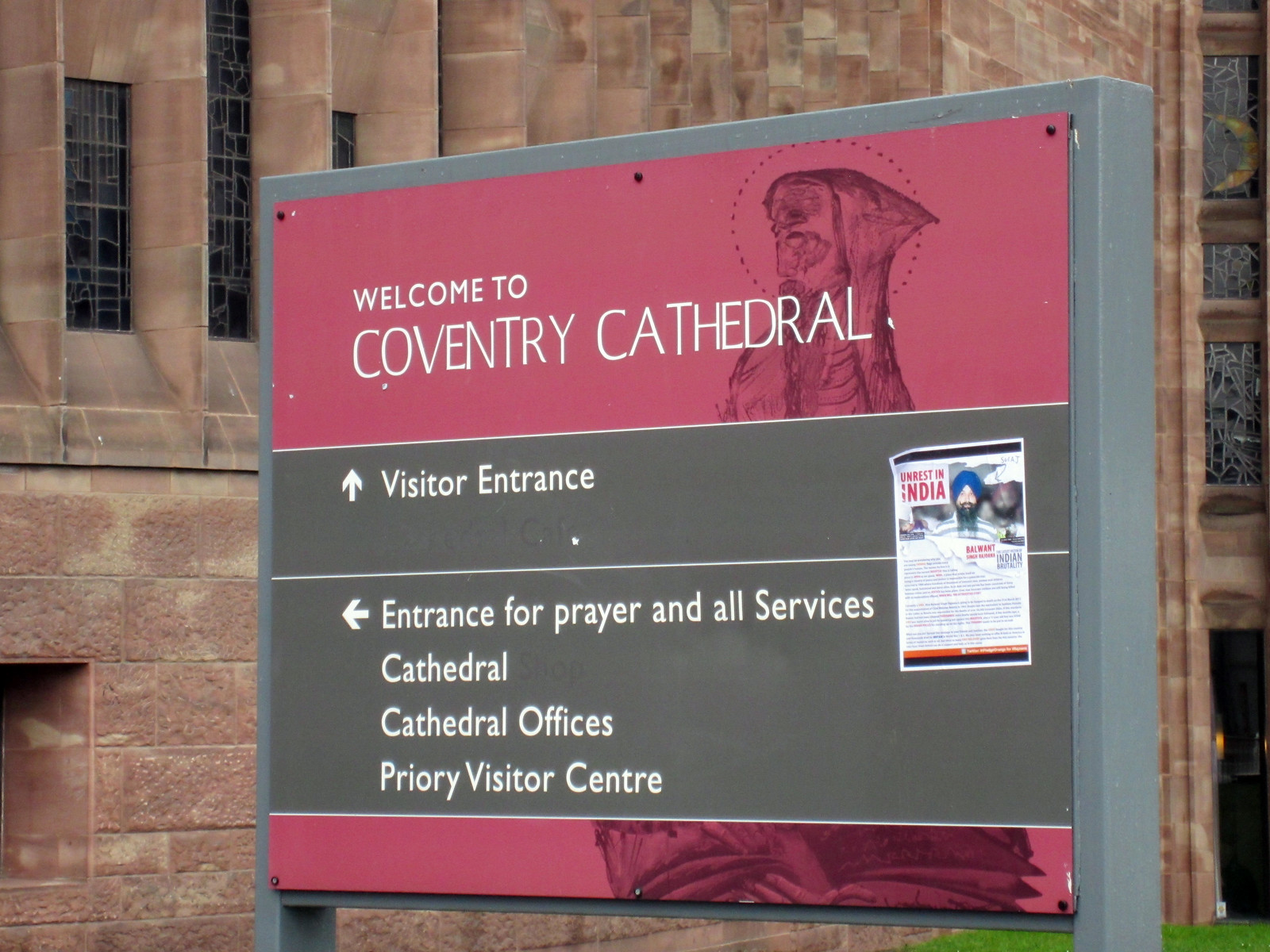The photograph showcases a detailed sign in front of a reddish-brown, ornately bricked building, which features a few small stained glass windows. The building, identified as Coventry Cathedral, is hinted at having a door in the bottom right corner, leading into a dark interior space. The sign prominently features two colored sections: a red banner at the top with white lettering that states "Welcome to Coventry Cathedral," and below it, a gray banner indicating directions. 

In the gray section, the text reads "Visitor Entrance" with an arrow pointing up, and underneath it, another arrow pointing left with the words "Entrance for Prayer and All Services, Cathedral, Cathedral Offices, Priory Visitor Center." The sign also includes an artistic sketch likely depicting a priest, indicated by a dotted line resembling a halo around the head, adding an intriguing visual element. Additionally, there is a piece of paper, possibly taped to the sign, displaying a headline with mentions of "Unrest in India," drawing attention to an external issue. The overall impression is an inviting yet complex and detailed entrance notice for visitors to Coventry Cathedral.